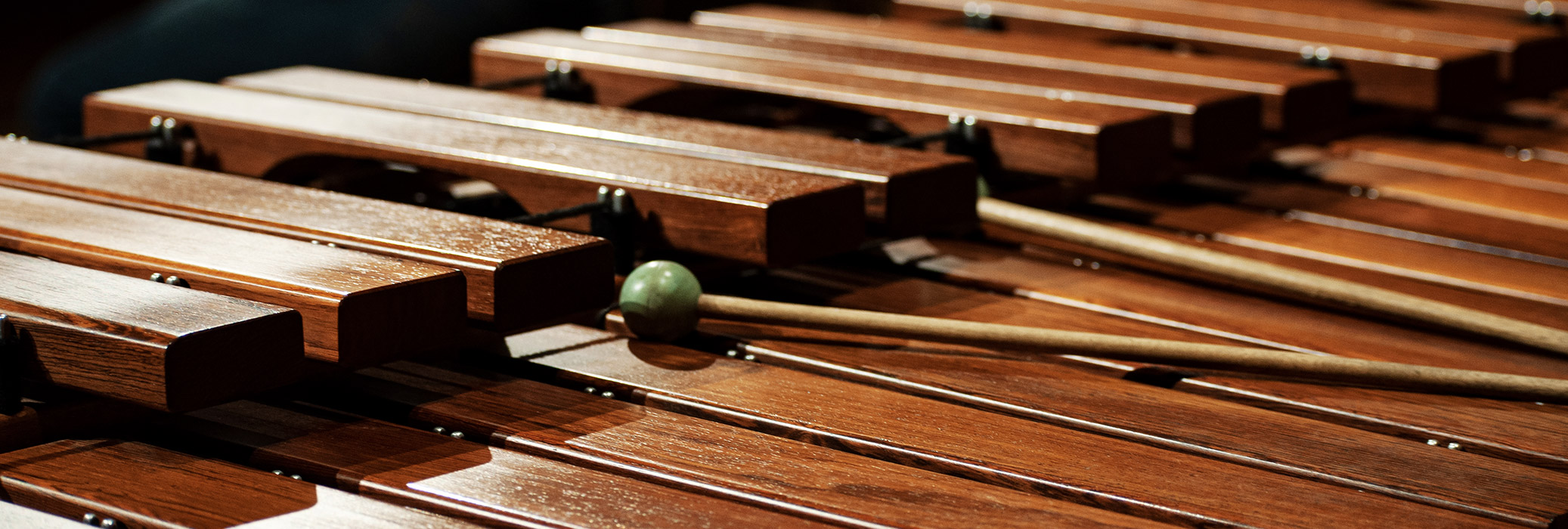This is a professional close-up photograph of a musical instrument, likely a xylophone or glockenspiel, featuring brown wooden bars arranged in two layers, with the upper layer slightly elevated above the lower one. The bars are shiny, dark, and reminiscent of redwood or polished park bench slats. Resting on the lower layer are two percussion mallets, each with a green rubber ball at the end of a narrow wooden dowel stick. The image, captured in a wide landscape orientation, shows the left side of the instrument in more detail while the right side fades into the background. The background in the top right corner is pure darkness, and the light focused on the instrument highlights its finely crafted details, emphasizing the professional quality of the photograph. There is no text on the image.